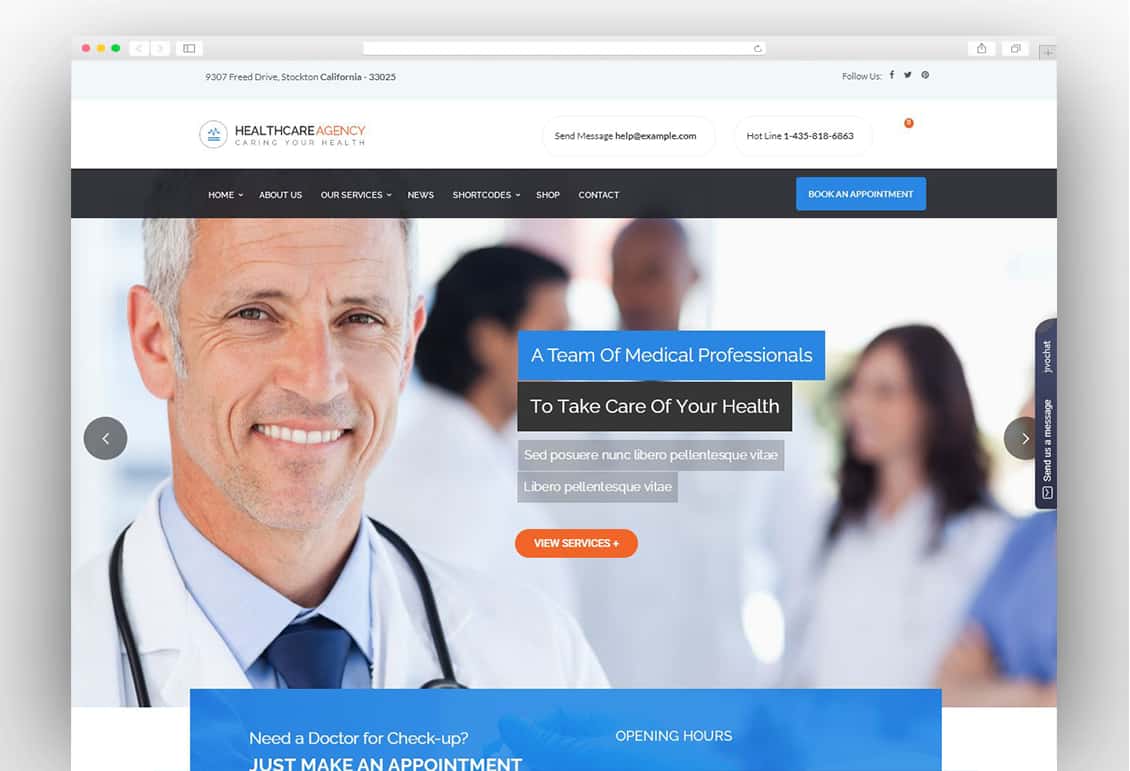This is a screenshot from a healthcare agency's website. At the top, the agency’s logo is prominently displayed within a brown circle. The logo features a rectangular box with a vertical stick flanked by two leaves on either side, symbolizing care and growth. Below the logo, the text reads: "Health Care Agency, Caring Your Health." 

On the right side of the screen, there is an option to send messages, with a contact email provided: help@example.com. Additionally, a hotline phone number is listed for immediate assistance. Across the top of the screen, a black navigation bar includes links to different sections of the website: Home, About Us, Our Services, News, Short Codes, Shop, and Contact. On the right side of this bar, there is a blue button labeled "Book an Appointment."

A prominently featured photograph shows an elderly gentleman with gray hair, standing confidently with a stethoscope around his neck. He is dressed in a white coat over a blue button-down shirt and a matching blue tie. He is smiling warmly, his brown eyes exuding kindness. His hair is neatly trimmed, reaching down to almost the end of his ears.

Beneath his picture, a blue box contains the text: "A Team of Medical Professionals," followed by a black box with the phrase: "To Take Care of Your Health." These phrases are also displayed in Spanish below. An orange box underneath invites users to "View Services."